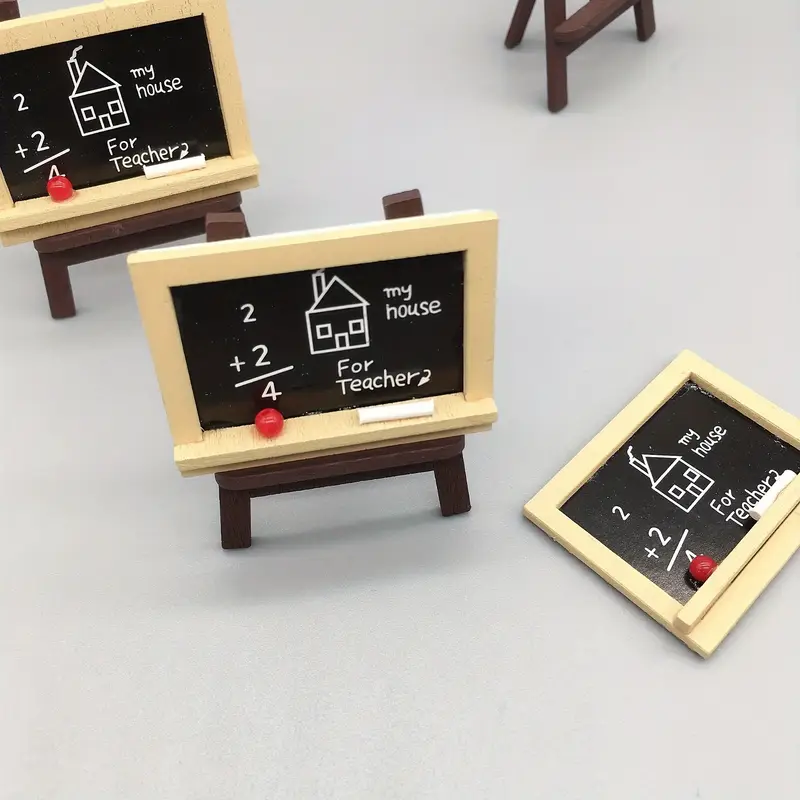The photograph showcases a group of miniature novelty chalkboards arranged on brown wooden easels. The image has a rectangular format, slightly longer on the left and right sides than the top and bottom. There are four easels in total, three of which hold identical chalkboards, while the fourth easel, located in the top right corner, is empty. The central chalkboard and the one to its top-left are positioned upright, while another identical chalkboard lays flat on what appears to be a gray floor.

Each chalkboard features a light brown wooden frame with a small ledge at the bottom. Resting on the ledge are a diminutive white cylindrical piece representing chalk and a round red plastic ball symbolizing an apple. The chalkboard surface is a black sticker adorned with white text and illustrations. The text reads, "2 + 2 = 4" along with an outline of a house labeled "my house," followed by the words "for teacher" and an arrow pointing towards the house. These miniature blackboards seemingly serve as novelty decorations, possibly intended for classroom use as playful aids rather than functional writing surfaces.